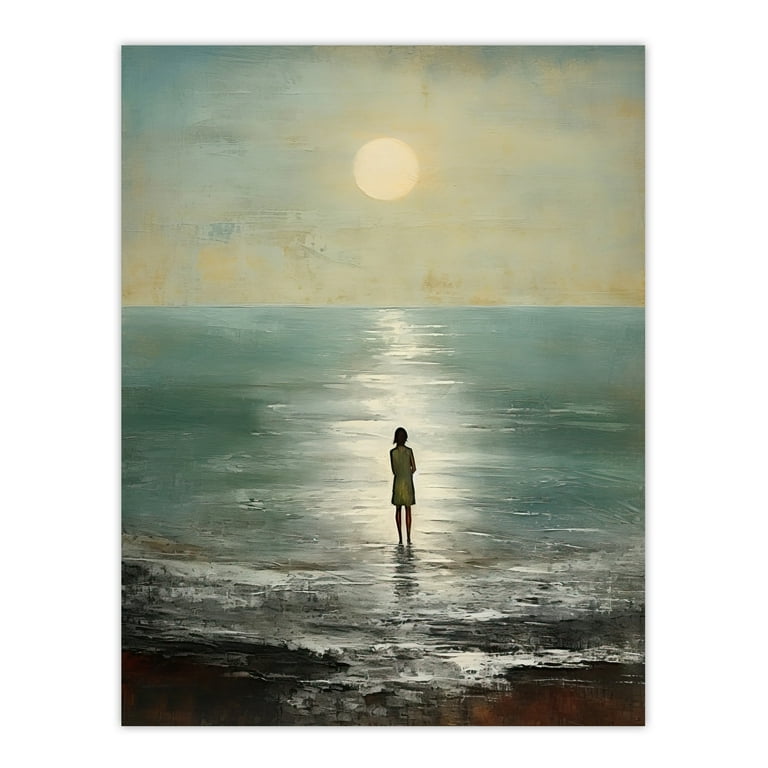The painting depicts a serene scene at the edge of a sea, emphasizing the tranquil interplay between sky, water, and a solitary female figure. The woman, viewed from behind, stands at the shoreline, her feet immersed in the gentle, blue waves. She is dressed in a green dress with long sleeves that extends just above her knees, and her hair falls gracefully around her neck. The sky, occupying about a third of the canvas, is a mesmerizing blend of bluish gold and hints of orange, dominated by a pale yellow orb representing either the sun or the moon. This celestial body casts a soft, white-gold light, which streaks elegantly across the water's surface, creating a luminous path. The waves exhibit subtle white caps as they approach the brown sand of the shore, emphasizing the natural colors and textures. The overall palette of the painting is composed of shades of blue, brown, and gold, creating an ethereal and peaceful ambiance with no other elements disturbing this tranquil setting.